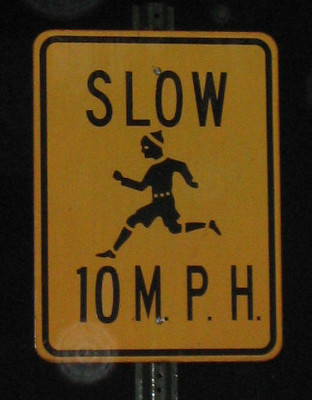The image captures a rectangular road sign mounted on a metal post, primarily occupying the frame. The sign is a distinct light orange or yellowish color with a thin black border just inside its rounded edges. Centered at the top of the sign, the word "SLOW" is prominently displayed in capital letters in black print. Below this, there is a black silhouette of a person running to the left, characterized with details resembling an elf, such as a pointy hat and small dots around the waist, mimicking a belt. This whimsical figure suggests an "elf crossing." Beneath the running figure, the text "10 M.P.H." indicates a speed limit of 10 miles per hour. The overall quality of the image is low, and it appears to have been taken at night, as the background is very dark and blurry. This sign, with its clear markings and playful design, likely serves to alert drivers to slow down in areas where pedestrians, possibly children or themed as elves, may be crossing, making it a useful indicator in school zones or crosswalks for safety.